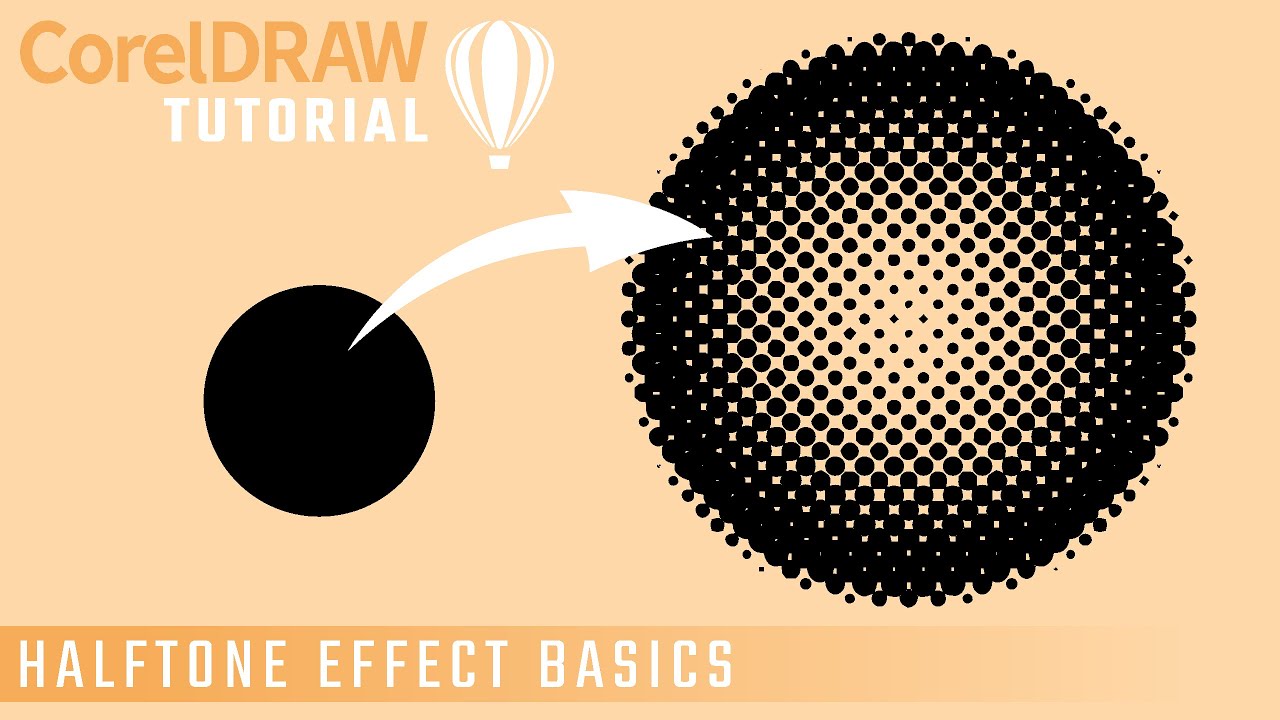The image is a detailed tutorial diagram featuring elements of CorelDRAW. At the top left, the word "CORELDRAW" appears in orange against a pink background, with "TUTORIAL" written below it in white letters. To the right, there's an outline sketch of a hot air balloon rendered in white. Below this, a prominent solid black circle has a white arrow arcing from its center to a larger, pixelated circle to its right. The larger circle displays numerous small dots that increase in size and density toward its perimeter, contrasting with a tan-yellowish background that becomes visible as the dots spread out. At the bottom left corner, a darker orange banner with an orange background sports the inscription "HALF TONE EFFECT BASICS" in white, capitalized text.